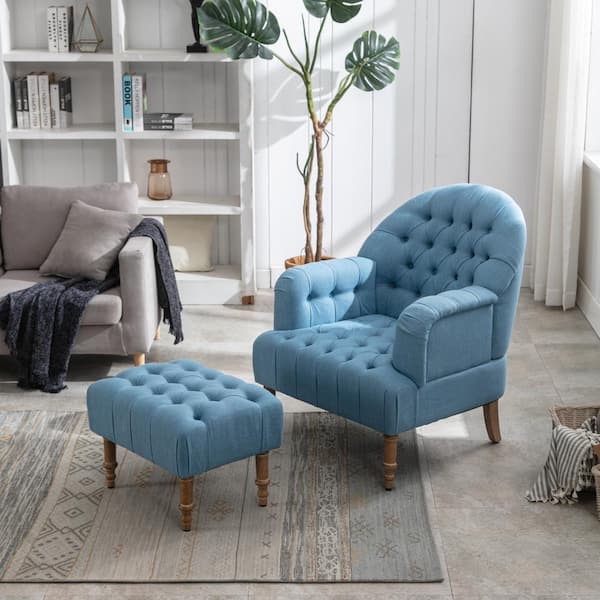The image portrays a cozy living room with a harmonious color scheme. Central to the scene is a light blue sofa accompanied by a matching blue ottoman, both supported by brown wooden legs with a similar design. The room features a gray, tile-like floor, softened by a carpet underneath the furniture. Directly behind the blue sofa, a tall plant with at least three large leaves adds a touch of nature. Adjacent to the blue sofa is a gray couch, partially visible, adorned with a black blanket. White walls and a white shelf in the background house an array of books and pots, contributing to the room's inviting and organized ambiance. A vent is noticeable on the side, and the room is illuminated by what seems to be a window on the right. The overall atmosphere is clean, detailed, and thoughtfully decorated.